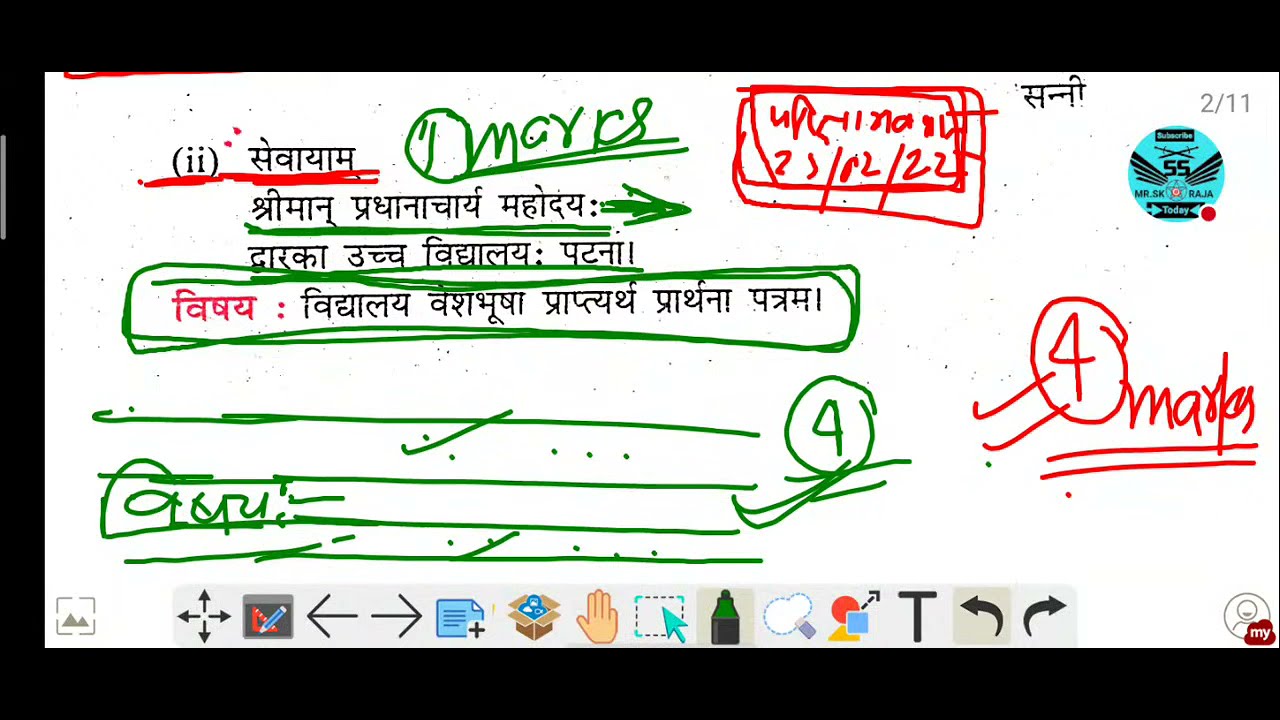The image depicts a horizontal rectangular screen of a hand-held electronic device, displaying a white interface with text in Arabic script. The screen is surrounded by a black border on the top, left, and bottom sides, with the right side border omitted. There are four primary lines of text, predominantly in black, except for one word on the bottom left which is highlighted in red. The first line of text also contains some red highlighting, while the second line is underlined in green, and the bottom line has a green border. Additional scribbles and potentially more lettering are visible underneath the main text, with two distinctive circled numbers: a green circled "4" and a red circled "4" with two red lines extending from the bottom. In the top right corner of the screen is a red-outlined box containing numbers and letters, adjacent to more black Arabic text and a gray "2-11". Beneath the main section of the screen is a toolbar with various icons resembling functions from a graphic or note-taking program, such as pen, select, text, arrow, copy, and movement tools, indicating that this image could be from some kind of graphic design or annotation application.